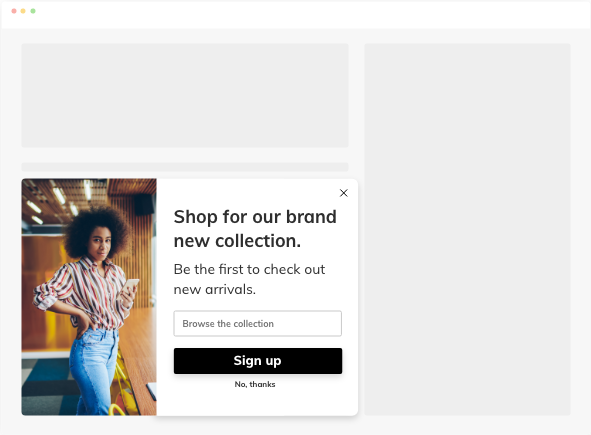At first glance, the image appears to be a screenshot of a web page, albeit with incomplete information. The backdrop is notably blank, accentuating a lone square section located in the bottom left corner. This section features a photograph of an African American woman with a natural, bushy brown afro. She exudes confidence in a vertically striped shirt featuring red, white, and black hues, with the sleeves rolled up to her elbows. Her right hand rests authoritatively on her hip, while her left hand holds a light-colored phone, potentially light gold or gray, though its precise color is indecipherable due to some blurriness.

The woman is dressed in light blue jeans and gives a cheerful, albeit closed-mouth smile. The background behind her consists of a brown wooden wall and flooring that combines tones of blue, black, and gray. Positioned to her right is a wooden table accompanied by yellow chairs, contributing a splash of color to the setting.

The informational content in the image includes a promotional message that reads, "Shop for our brand new collection. Be the first to check out new arrivals." Below this text, there's a button labeled "Browse the collection," next to a black rectangular button that says "Sign up." Below the "Sign up" button, in smaller black font, is a discreet "No thanks" option.

An adjacent gray rectangle situated above the information, and a larger vertical gray rectangle to its right, appear devoid of content, suggesting that additional details or images were intended but are conspicuously missing, lending an incomplete and somewhat sparse look to the overall web page design.